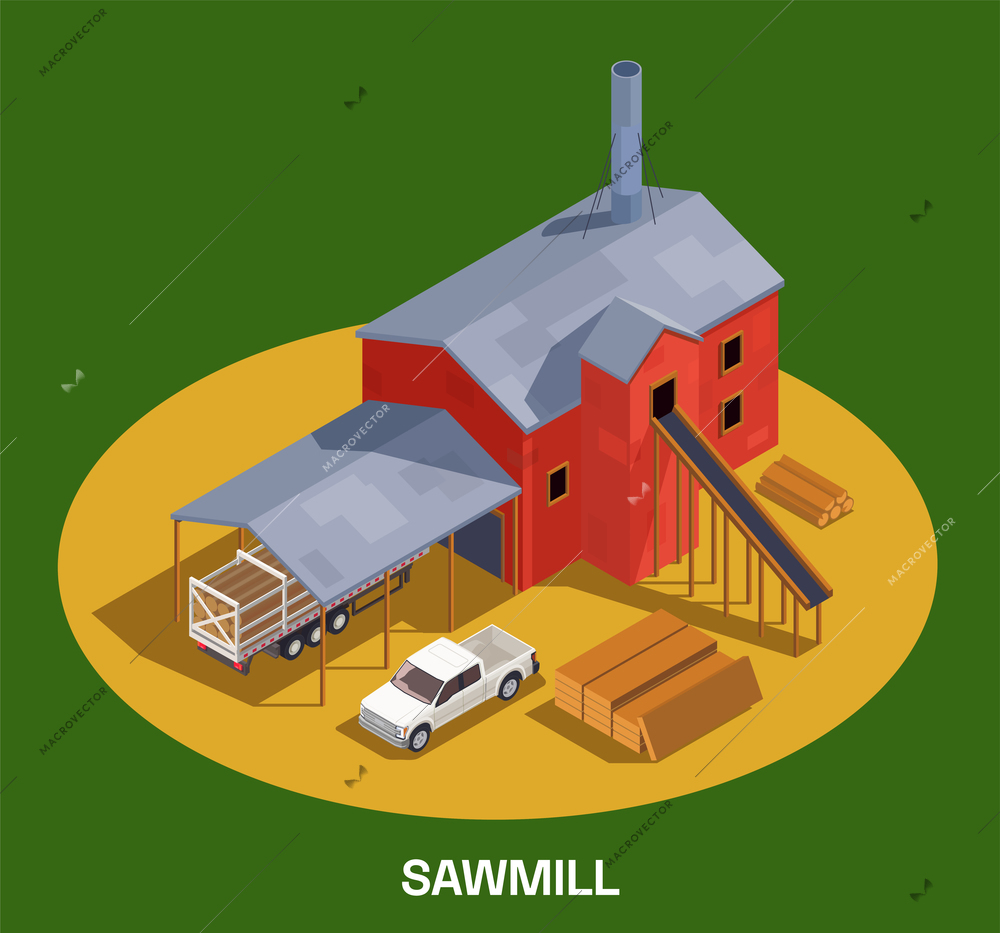The image is a digitally created representation of a sawmill centered in a solid green background. A noticeable watermark reading "Macrovector" spans across the screen, with the word "Sawmill" clearly marked at the bottom in white. The focal point is a red barn-like building positioned in the center, distinguished by its gray, silver-topped roof and tall chimney. The building features a conveyor chute extending from the second-floor window and a carport to the side. Below the barn is a white truck facing the bottom left corner, its bed empty. Surrounding the barn and scattered mainly in front are multiple stacks of lumber in various shades of brown. Adjacent to the truck is another set of logs. The digital illustration uses a palette of green, yellow, gray, white, and brown hues, effectively capturing the essence of a traditional sawmill.